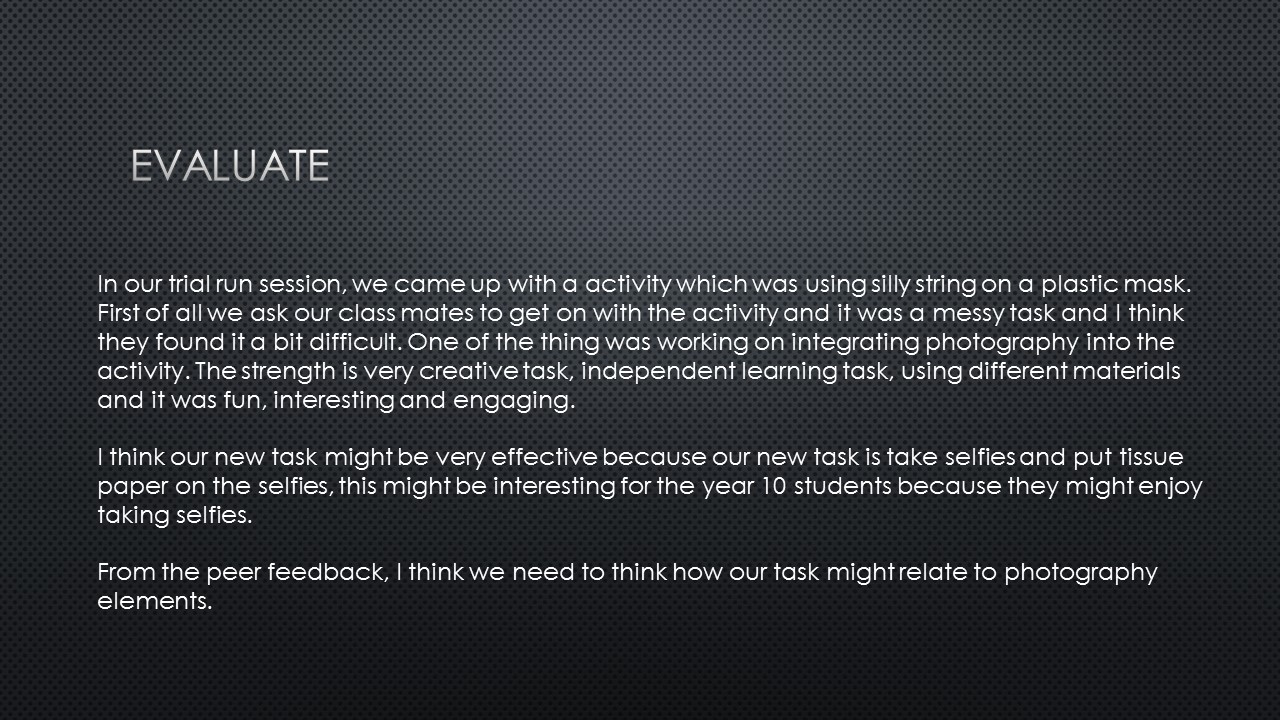The image showcases a PowerPoint slide with a black background and silver, white text. The header "EVALUATE" is prominently displayed in capital letters. Below the header, a detailed account describes a classroom trial run where students engaged in a creative and messy task using silly string on plastic masks. The activity, which aimed to integrate photography, was found to be somewhat difficult but highly engaging, fostering independent learning through the use of different materials. Peer feedback highlighted the task's fun and interesting nature. Additionally, a proposed new task involves taking selfies and decorating them with tissue paper, aiming to captivate Year 10 students by blending photography elements into the experience.